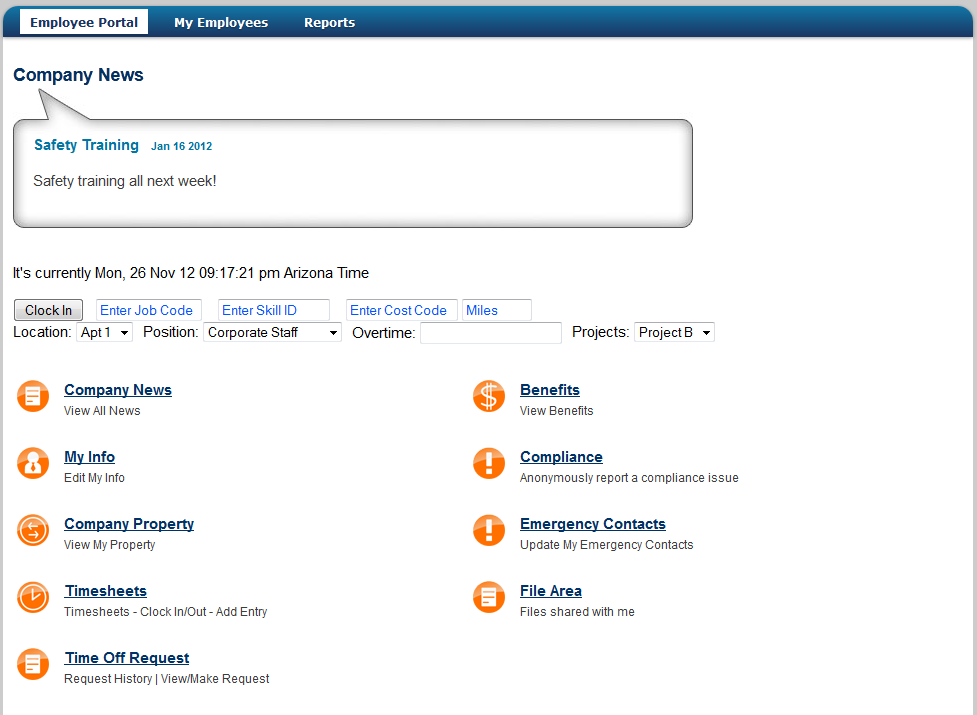The image depicts a computer screen with a detailed interface layout. At the top, there's a very thin gray border, slightly visible, that extends down the left and right sides but even thinner. Below this top edge is a dark blue area. On the left side of this dark blue section, there's a white horizontal rectangle with the text "Employee Portal" in blue font.

Beneath the dark blue header, on the right side, white font against the dark blue background displays the options "My Employees" and "Reports." Moving down to the main white background, "Company News" is written in bolded navy font. A speech bubble extends from "Company News," creating a horizontal rectangular area with "Safety Training" in turquoise font inside it, followed by the date "January 16, 2012" in black font and the message "Safety training all next week."

Outside this bubble, on the standard white background, it displays the current date and time in navy font: "It's currently Monday, 26 NOV 12:09:17:21 pm Arizona time." Below, there are several horizontal buttons. The first button is light gray with the text "Clock In" in black font. The remaining buttons are white with bright blue font and read: "Enter Job Code," "Enter Skill ID," "Enter Cost Code," and "Miles."

Further down, it says "Location:" followed by a pull-down menu showing "APT-1," then "Position:" with a pull-down menu displaying "Corporate Staff," "Overtime:" which is blank, and "Projects:" with a pull-down menu showing "Project B."

On the left column under dark blue bolded headlines, each underlined and accompanied by orange icon circles with white illustrations inside, are:

1. **Company News**  
   - View All News (orange circle with a white vertical paper icon)
2. **My Info** (blue)  
   - Edit My Info (black, with an icon of a person in an orange circle)
3. **Company Property** (blue)  
   - View My Property (black, with an icon of left and right arrows in an orange circle)
4. **Timesheets** (blue)  
   - Timesheets - Clock In/Out  
   - Add Entry (black, with a clock icon in an orange circle)
5. **Time Off Request** (blue)  
   - Request History  
   - View/Make Request (black, with a white paper icon in an orange circle)

In the second column, the sections are:

1. **Benefits** (blue)  
   - View Benefits (black, with a white dollar sign icon in an orange circle)
2. **Compliance** (blue)  
   - Anonymously Report a Compliance Issue (black, with a white exclamation point icon in an orange circle)
3. **Emergency Contacts** (blue)  
   - Update My Emergency Contacts (black, with a white exclamation point icon in an orange circle)
4. **File Area** (blue)  
   - File Shared With Me (black, with a white paper icon in an orange circle)

This detailed layout highlights various functional areas and features within the employee portal, each section identified by clear headings and corresponding icons.